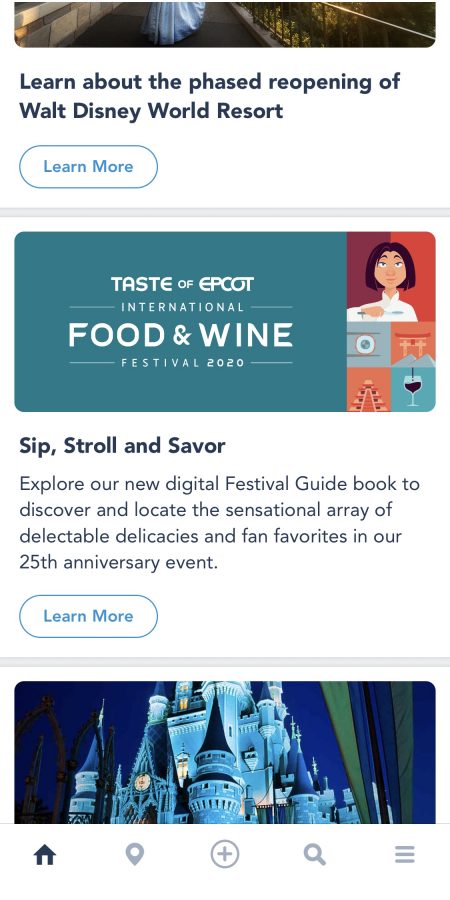This cell phone image captures a section of an online article about the phased reopening of Walt Disney World Resort. The upper-left corner showcases text that invites readers to "Learn about the phased reopening of Walt Disney World Resort," and the image partially displays the bottom of a princess gown against a luxurious stairwell with ornate railing details, exuding a sense of elegance and grandeur.

Below this, another segment introduces the "Taste of Epcot International Food and Wine Festival 2020." The visual element here resembles a credit card, featuring an illustration of a chef, wine, and various foods amidst vibrant colors, emphasizing the event's culinary delights. Accompanying this is a description: "Sip, stroll and savor. Explore our new digital festive guidebook to discover and locate the sensational array of delectable delicacies and fan favorites in our 25th anniversary event," along with a "Learn More" button to entice further exploration.

The bottom section of the image portrays a photograph of Cinderella's Castle, magnificently illuminated in blue hues. The perspective is from ground level, capturing the castle's intricate architecture and detailed windows. Although the topmost spires are not visible, the image beautifully showcases the structural elegance and enchanting design of this iconic Disney landmark.